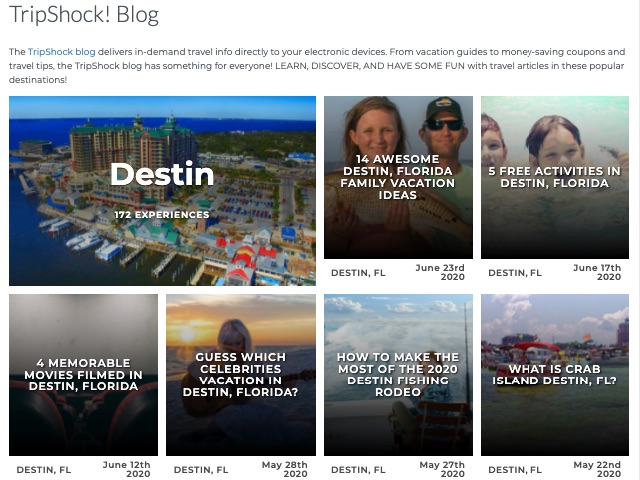This photograph showcases the front page of the TripShock Blog, displayed in landscape orientation against a white background. A thin vertical line on the right side serves as the only border element.

Prominently, the top left corner features the blog's header, "TripShock Blog," with the exclamation point emphasizing the word "shock." Directly beneath, in smaller font, is a brief tagline: "TripShock delivers in-demand travel info directly to your electronic devices—from vacation guides to money-saving coupons and travel tips. The TripShock Blog has something for everyone. Learn, discover, and have some fun with travel articles in these popular destinations."

Below this introductory section are visual links to various articles, organized into two rows. The top row comprises three images, each with a descriptive heading. The first image is an aerial view of a city by the water, accompanied by the text "Destin, 172 experiences." Adjacent to this, separated by a white border, is a picture of a man and woman titled "14 Austin Destin, Florida Family Vacation Ideas." The final image in the top row shows two children in a pool, labeled "5 Free Activities in Destin, Florida."

The second row features four more images with corresponding descriptions. The first highlights "Four Memorable Movies Filmed in Destin, Florida." Next is an article entitled "Guess What Celebrities Vacation in Destin, Florida," followed by "How to Make the Most of the 2020 Destin Fishing Rodeo." The final image addresses the question, "What is Crab Island in Destin, Florida?"

Each article is visually represented, inviting readers to explore various aspects of traveling to Destin, Florida, through engaging and informative content.